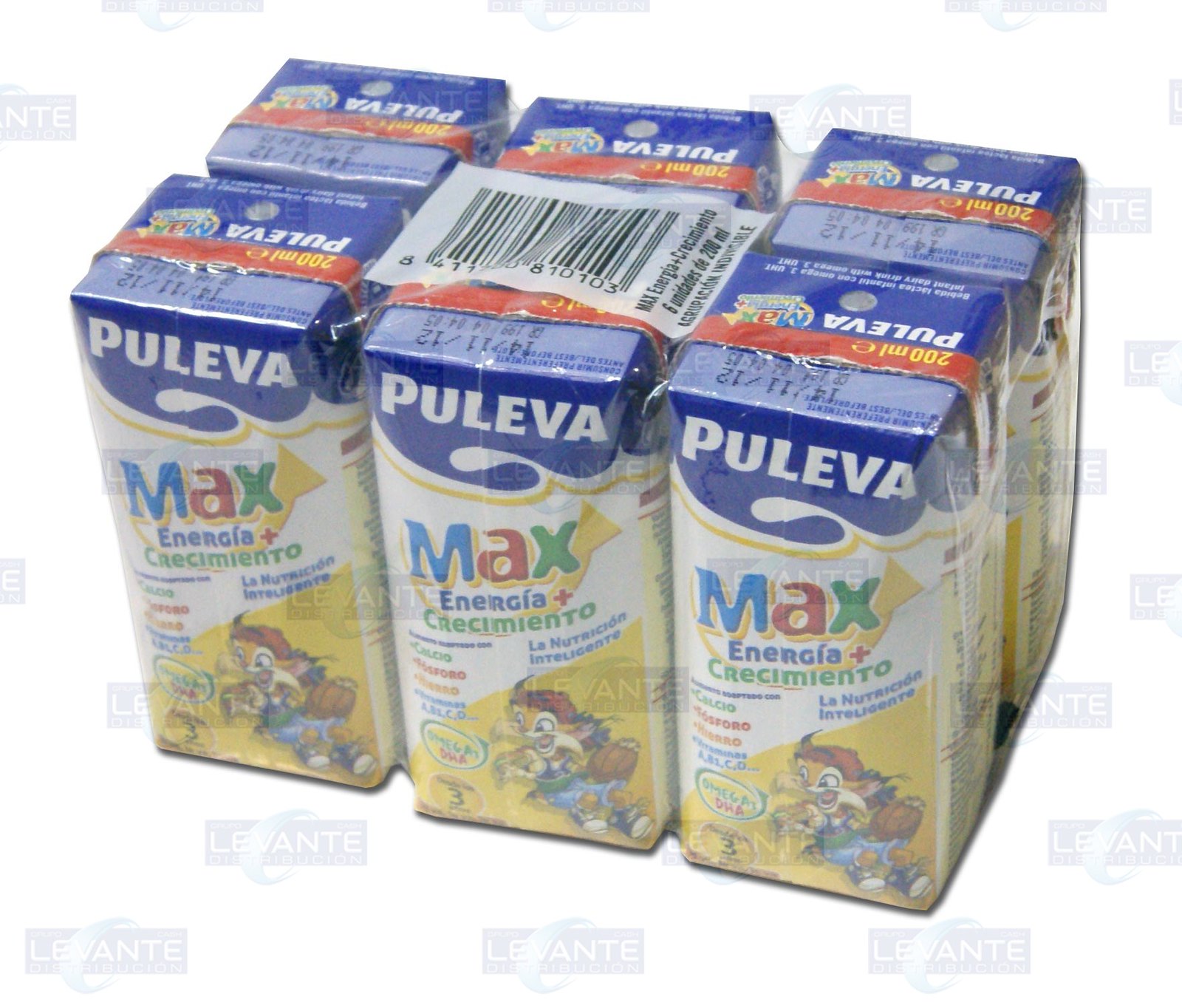This is a detailed product image of a six-pack of Spanish juice boxes or nutritional supplement drinks. The six-pack is fully wrapped in supermarket plastic, with a barcode printed on the top. Each juice carton prominently features the brand name "Pulevo" in bold white letters against a blue background at the top. Below this, against a diagonally divided yellow and white background, there’s a colorful illustration of an anthropomorphized cartoon animal, possibly a fox or bobcat, donning a red backwards baseball cap, green t-shirt, and jeans, holding a basketball and smiling energetically. The text "Max Energia plus Crecimiento" is seen on each box, indicating that the drink is likely energy-boosting and growth-promoting, targeted towards children. The image is faintly overlaid with repeating watermarks that potentially say "Levante" or "Galvante," making it discernible as a promotional or stock photo.